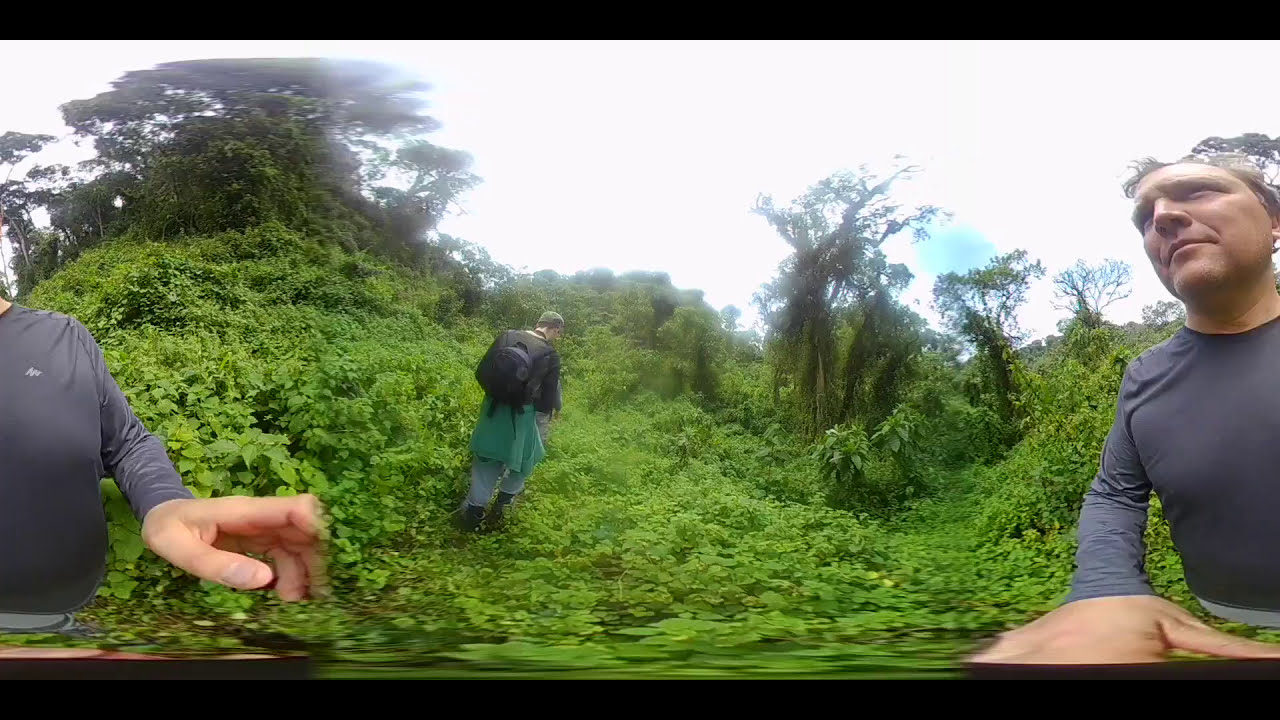In this photograph, we see two individuals navigating through a dense, lush jungle. The ground is vibrant with green plants, and sporadic trees are seen on the sides. Dominating the center of the image is a man, captured from the back, wearing a black jacket, white pants, and a black backpack. He is walking away from the camera, seemingly on a trail. The person taking the picture, visible on the right, wears a dark gray long-sleeve shirt. The photo has a panoramic, fisheye effect, curving the image and splitting it into two. Above, the sky appears bright white, indicating daylight. These two men, engaged in their hike, showcase the wild and verdant atmosphere of the jungle.